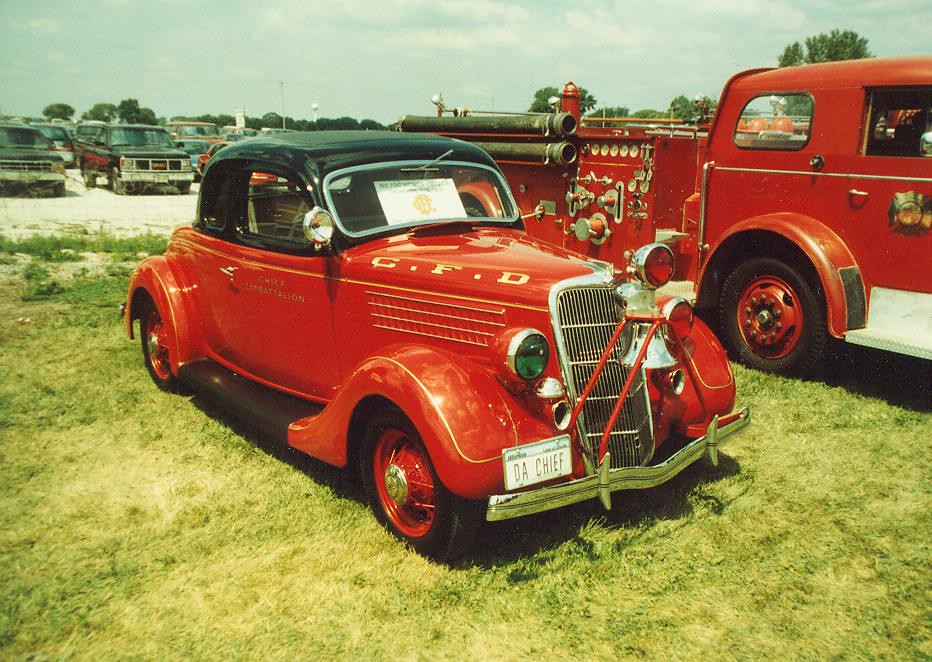A nostalgically atmospheric horizontal image captures a scene from an antique car and service vehicle show, showcasing a beautifully preserved late 1940s fire chief's car alongside a vintage 1950s fire truck. The image, yellowed with age, tells a story of yesteryear's emergency response vehicles. 

The fire chief's car, a striking hardtop coupe, features an Illinois license plate reading "DA CHIEF." Adorned with gold-lettered "CFD" on its hood, possibly denoting the Chicago Fire Department, the vehicle's design is meticulously detailed with a red lower body contrasted by a black top. Chrome handles accentuate the doors, bumpers, and windshield frame, while a mounted bell and a red light at the very front evoke an era of distinctive, hands-on firefighting.

Beside it stands the robust and commanding presence of a 1950s fire truck. Displaying a gold shield on its door, this water pumper or cannon truck is equipped with an array of pipes, hoses, gauges, and valves, essential for combating fires. Both vehicles are oriented towards the right-hand side of the image, resting on lush green grass. The background reveals a gravel parking lot filled with pickup trucks, adding to the nostalgic charm and authenticity of the scene.

This image not only documents the impressive machinery of a bygone era but also captures the spirit and dedication of historic fire departments.